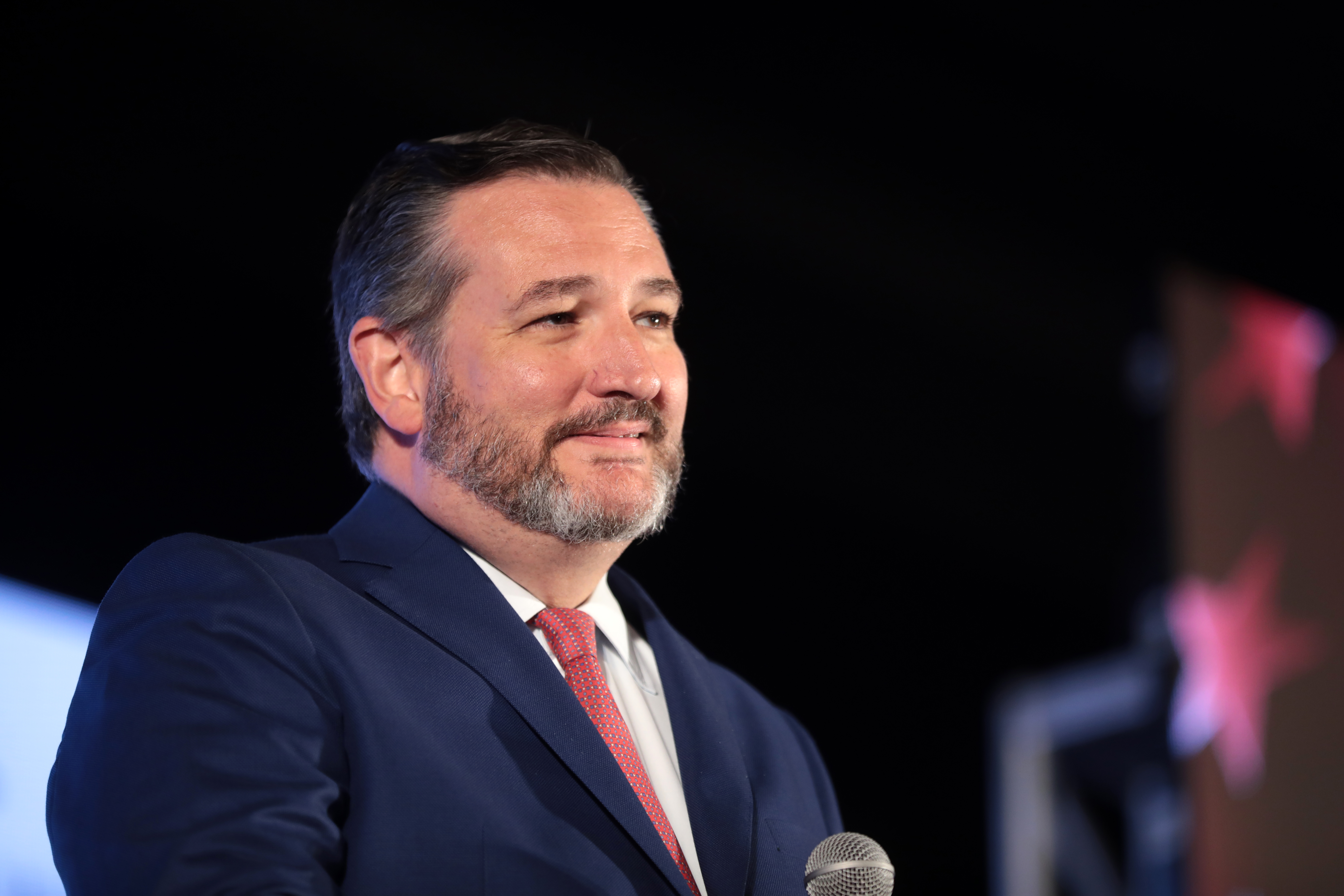In this detailed photo of Ted Cruz, the U.S. Senator from Texas, he is depicted as a light-skinned man with short, dark hair speckled with some gray. He sports a neatly trimmed beard and mustache that also exhibit strands of gray. Ted Cruz is dressed in a dark blue suit paired with a white button-up shirt and a tie that is predominantly red with subtle white and blue dots. He appears to be in mid-speech, holding a microphone at chest level, which suggests he could be at a podium, possibly addressing an audience or participating in a forum. His facial expression includes a smile with eyes half open, indicating he might be engaging with someone off-camera. The background is predominantly black, enhancing the focus on Cruz, and features a blurred section on the right with white stars against a red flag, common to political events like CPAC. The backdrop includes some brightly colored signs and possible light displays, further suggesting he is on a stage under a spotlight.